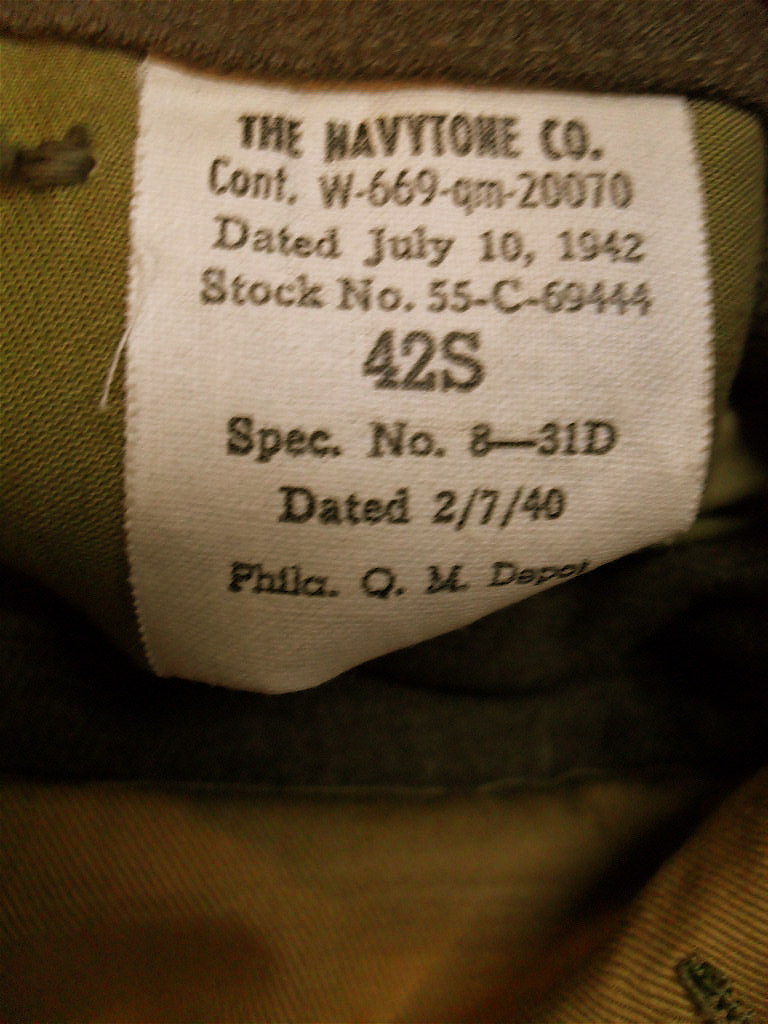This image displays a close-up view of a label sewn onto a piece of fabric, likely part of an army uniform. The label is square-shaped, white, with black lettering. It reads "The Havitone Company," followed by "Cont W-669-Q-M-20070." The label is dated "July 1942" with a stock number "55-C-69444." Additionally, it indicates a size "42-S," a specification number "8-31-D," and another date "2-7-1940." The label also references "Philadelphia, Q-M Depot." The background fabric has a tannish-green hue, suggestive of military attire. The label appears to be situated on the inside of a collar. At the bottom right-hand corner of the image, a buttonhole is visible, stitched with thread matching the army green color of the fabric.